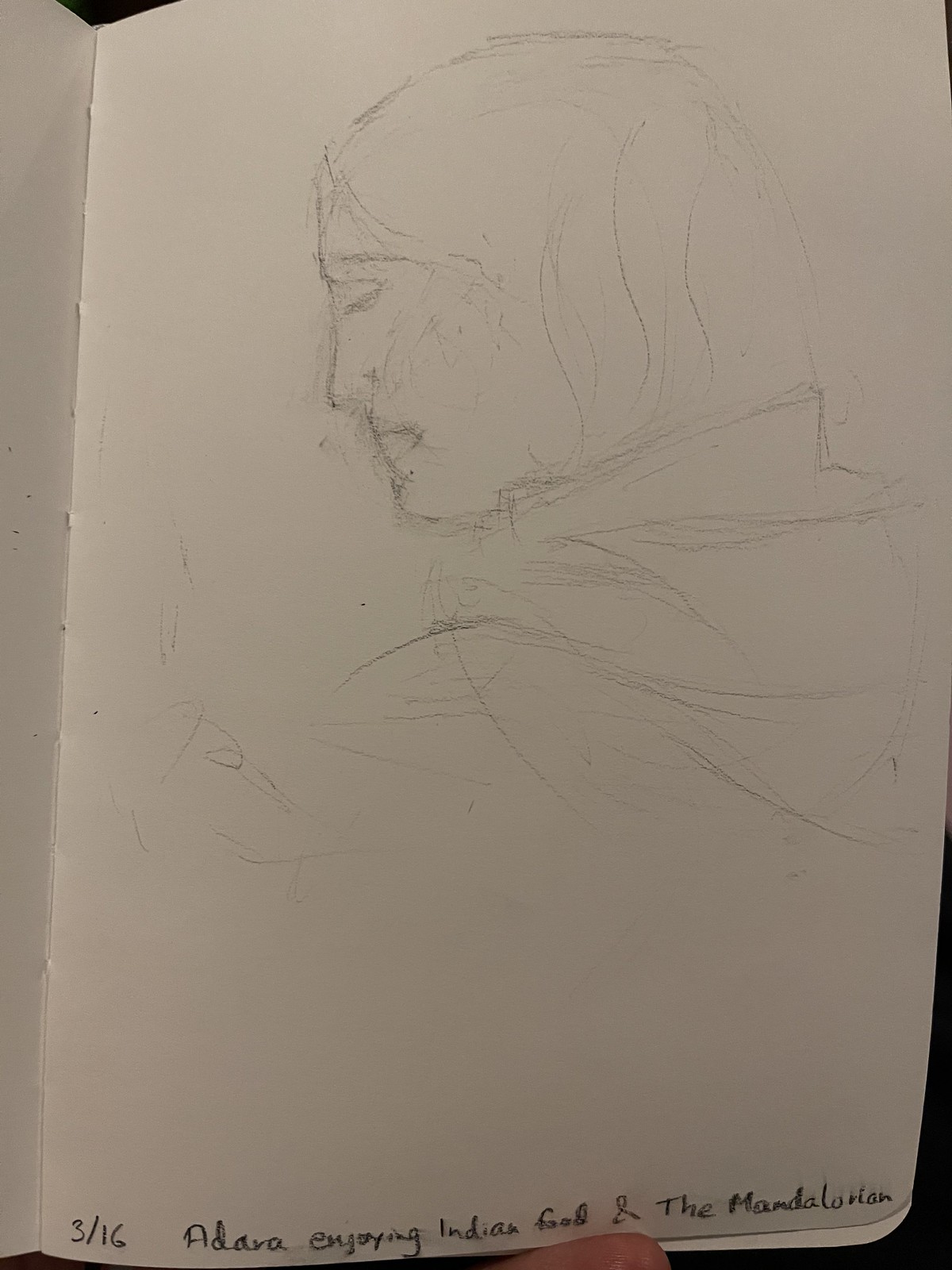This pencil drawing on paper depicts a left side profile of a woman with her chin tilted down towards her chest, embodying an aura of melancholy and disappointment. Her closed eyes and gently downturned mouth express a palpable sense of sorrow. The image, rendered entirely in black and white, focuses on the emotional depth of the subject rather than intricate details like her hair, which remains undefined. The minimalist use of pencil on paper serves to intensify the poignant expression captured in this somber portrait.